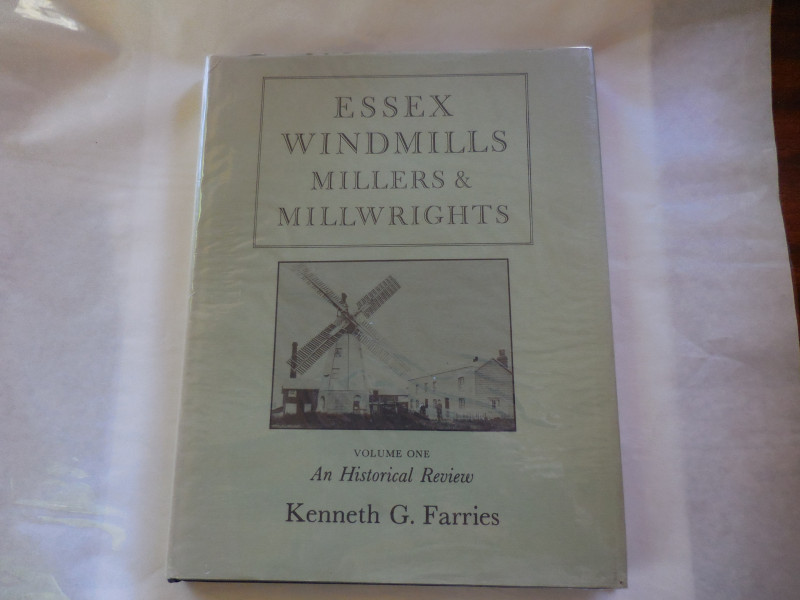The image features a book presented on a white sheet, possibly tissue or wrapping paper, covering a table. The book, a pale green volume titled "Essex Windmills, Millers, and Millwrights: Volume 1, An Historical Review" by Kenneth D. Farries, dominates the scene. The cover design includes a black rectangle at the top with the title's words stacked sequentially, followed by a black and white photograph of a large windmill accompanied by an adjacent building. Below this image, additional text reads "Volume 1" in uppercase, "An Historical Review" in italics, and "Kenneth D. Farries" in larger font. The focus of the image is solely on this historical book, with no other objects or colors present.